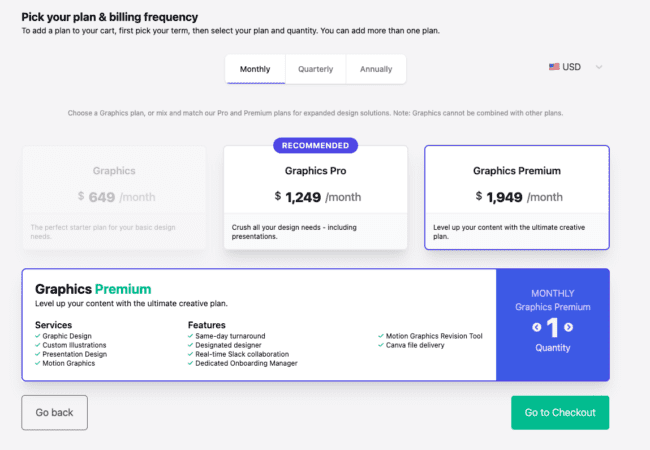The image features a detailed user interface for selecting a subscription plan, with the title "Pick your plan and billing frequency" in black text in the upper left corner. Below this, in smaller text, it instructs users to choose their team and plan, indicating that multiple plans can be selected. Billing options—monthly, quarterly, and annually—are listed, with "monthly" highlighted in purple.

To the right, a small image of the American flag is displayed next to "USD," denoting the currency. Users are prompted to either select a graphics plan or combine professional and premium plans for enhanced design solutions, noting that graphics cannot be mixed with other plans.

The "Graphics" plan priced at $649 per month appears blurred out. In the center, a white square prominently showcases the "Graphics Pro" plan at $1,249 per month, marked as "Recommended." This plan claims to fulfill all design needs, including presentations. Below that, the "Graphics Premium" plan, outlined in a purple box and priced at $1,949 per month, is highlighted with "Premium" written in green. It promises to elevate content with top-tier creative services and features. 

Additionally, a purple box displays the "Monthly Graphics Premium" option with a default quantity of one. The interface concludes with a green rectangle in the bottom right corner labeled "Go to checkout."